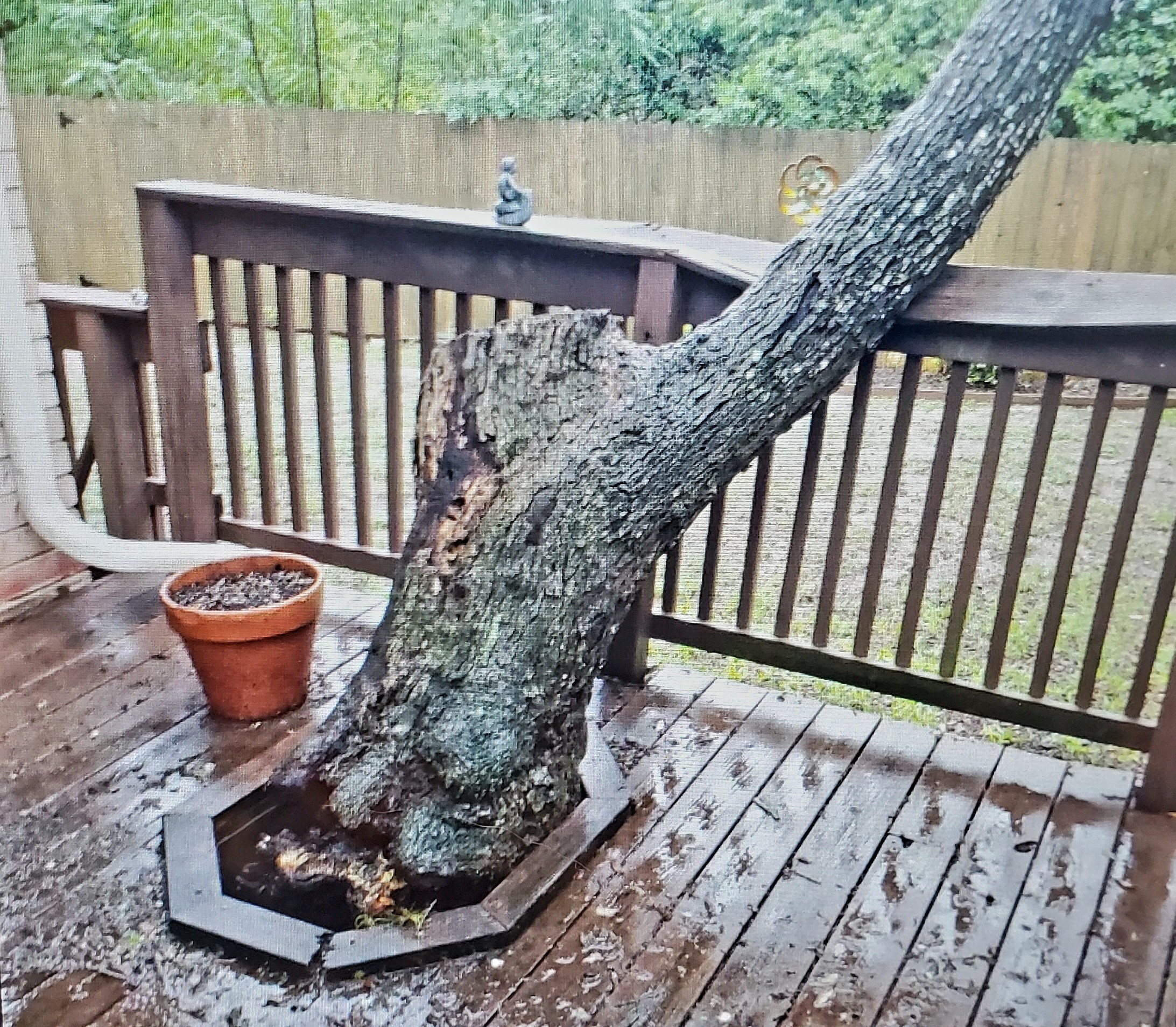Captured in broad daylight amidst a gentle rain shower, this photograph depicts a serene outdoor scene, likely in a backyard. The glistening wet surfaces enhance the vivid greenery and bring a fresh, rejuvenated look to the surroundings. In the background, a cluster of trees stands tall behind a classic wooden fence, contributing to the tranquil ambiance. The focal point of the image is a unique deck structure, ingeniously designed with a hole cut out to accommodate a lush, green, and sturdy tree growing through it. This blend of natural and man-made elements creates an enchanting visual. Adorning the deck's ledge are a charming clay pot and several garden ornaments, adding a touch of rustic garden aesthetics to the picturesque setting.